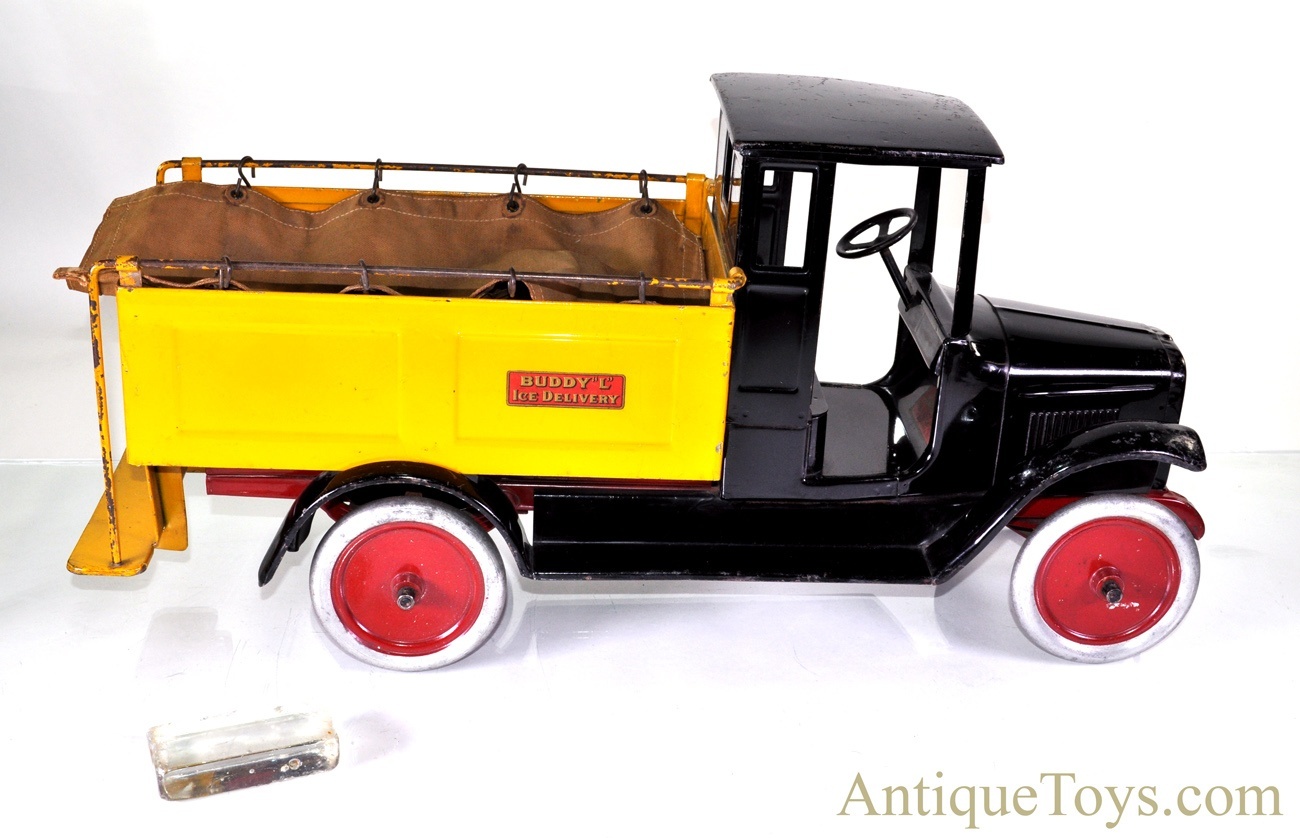The image features a detailed side profile of a die-cast antique toy truck, facing to the right. The main body of the truck is black, with a striking yellow truck bed that features a brown rack on the side. The text on the truck bed reads "Buddy's Ice Delivery." The toy truck has distinctive red wheels with white rims and lacks doors, showing an open steering wheel intended for standing operation. The vehicle appears to be designed without pedals or additional internal instruments, and it is missing a seat. The toy is set against a white background, likely indicating a professional photo shoot, and in the bottom right corner, it bears the website "Antiquetoys.com" in a light beige or goldish color. Additionally, a white rectangular prism, possibly representing ice, is visible at the bottom left of the image. This depiction showcases the intricate details and nostalgic design of an antique toy truck, emphasizing its vintage charm and craftsmanship.